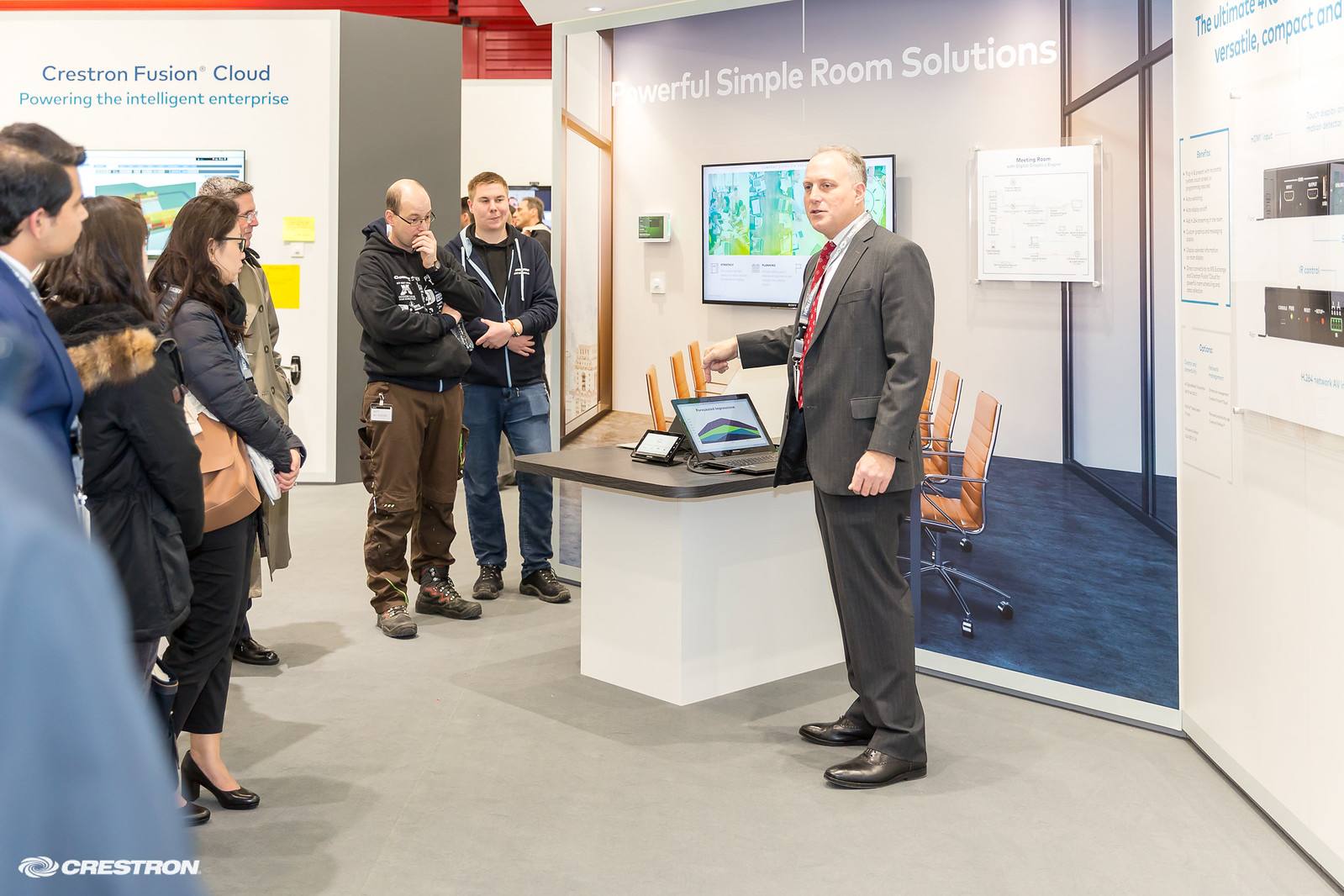The photo captures a scene inside an office building or large hallway, where a man is giving a presentation to a group of approximately six to eight people. The man, bald and dressed in a dark gray suit with a reddish tie, stands next to a small table or counter with a white base and black top, which holds an open laptop. He is positioned slightly towards the audience, primarily showing his left side, and points downwards as he speaks. The audience, attired casually in jeans, pants, long-sleeve shirts, and hoodies, listens intently.

Behind the man, a wall features a printed design of a conference room with white text reading "Powerful Simple Room Solutions" at the top. To the right of this is a section of white wall with a partially visible diagram and blue text, located in the upper corner of the image. On the far left side, another wall displays the words "Crestron Fusion Cloud powering the intelligent enterprise." The setting's light gray floors and paneled walls contribute to the modern, professional ambiance, with indoor lighting illuminating the scene and a hallway that extends further into the distance.